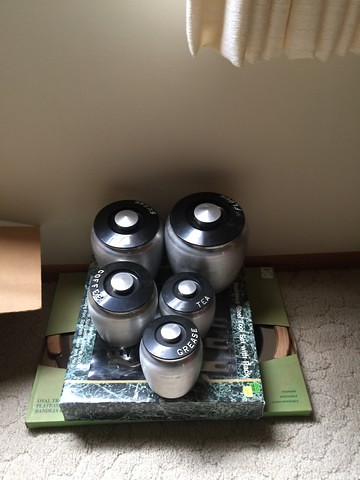In this indoor photograph, the scene features an off-white wall with matching off-white curtains visible in the upper right-hand corner, their fabric folds softly illuminated. The floor is covered in a plush, grayish-tan carpet. Positioned against the wall is a set of two books; the bottom book is green, and the top book has a distinctive bluish marble pattern. Resting atop these books are five stainless steel canisters, each with a black lid capped by a stainless steel knob. The canisters vary in size, from smallest to largest, and are typically used for storing kitchen essentials like flour, sugar, and spices. The middle row, left canister, is labeled "coffee," the right canister "tea," and the bottom canister is labeled "grease." The labels on the two canisters in the background are illegible. The arrangement creates a striking visual contrast against the neutral-toned background.